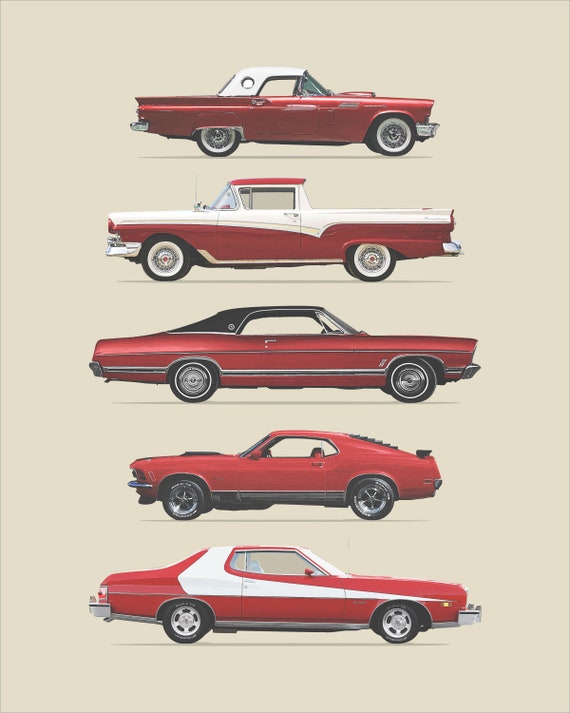The poster features hyper-realistic illustrations of five distinct Ford vehicles, aligned vertically against a cream-colored backdrop. All vehicles share a rich ruby red base with varying accent colors. 

At the top of the poster is a classic Ford Thunderbird from the 1950s or 60s, characterized by its two-door design, red body, and white convertible top with a small window. Below it is a Ford Ranchero, an older model truck with a red and white body and a red roof. The third car from the top is a Ford LDT, an older two-door sedan sporting a red body and a black vinyl top. The fourth vehicle is a Ford Mustang, a sporty hatchback with a red body and black louvers on the rear window. At the bottom of the poster is the iconic red Ford Torino from the 1970s, distinguished by a bold white stripe that starts on the passenger side and narrows as it extends toward the roof. The detailed portrayal and rich color palette of the cars highlight their classic appeal, with no accompanying text to distract from their visual impact.